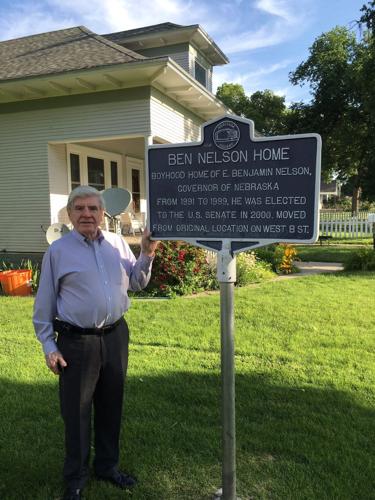This detailed photograph captures an elderly man, possibly E. Benjamin Nelson, standing in front of a historical marker that reads "Ben Nelson Home - Boyhood home of E. Benjamin Nelson, Governor of Nebraska from 1991 to 1999. He was elected to the U.S. Senate in 2000. Moved from original location on West 8th Street." The man, with gray hair, is dressed in a white button-down shirt, brown pants, and brown shoes, and he has one hand resting on the sign. The day is sunny with misty clouds in the sky, casting a pleasant light on the scene.

In the background, there is a well-kept lawn in front of a house with greenish-blue siding and a shingled roof. A tidy walkway leads up to the home, which is complemented by a picket fence and a cozy porch decorated with chairs, an orange tub, and a couple of satellite dishes. The house is surrounded by a neatly trimmed lawn and flower borders, adding to the overall charm of the location. Despite not smiling, the man appears content and proud to stand by this historical marker, commemorating his significant contributions and legacy.